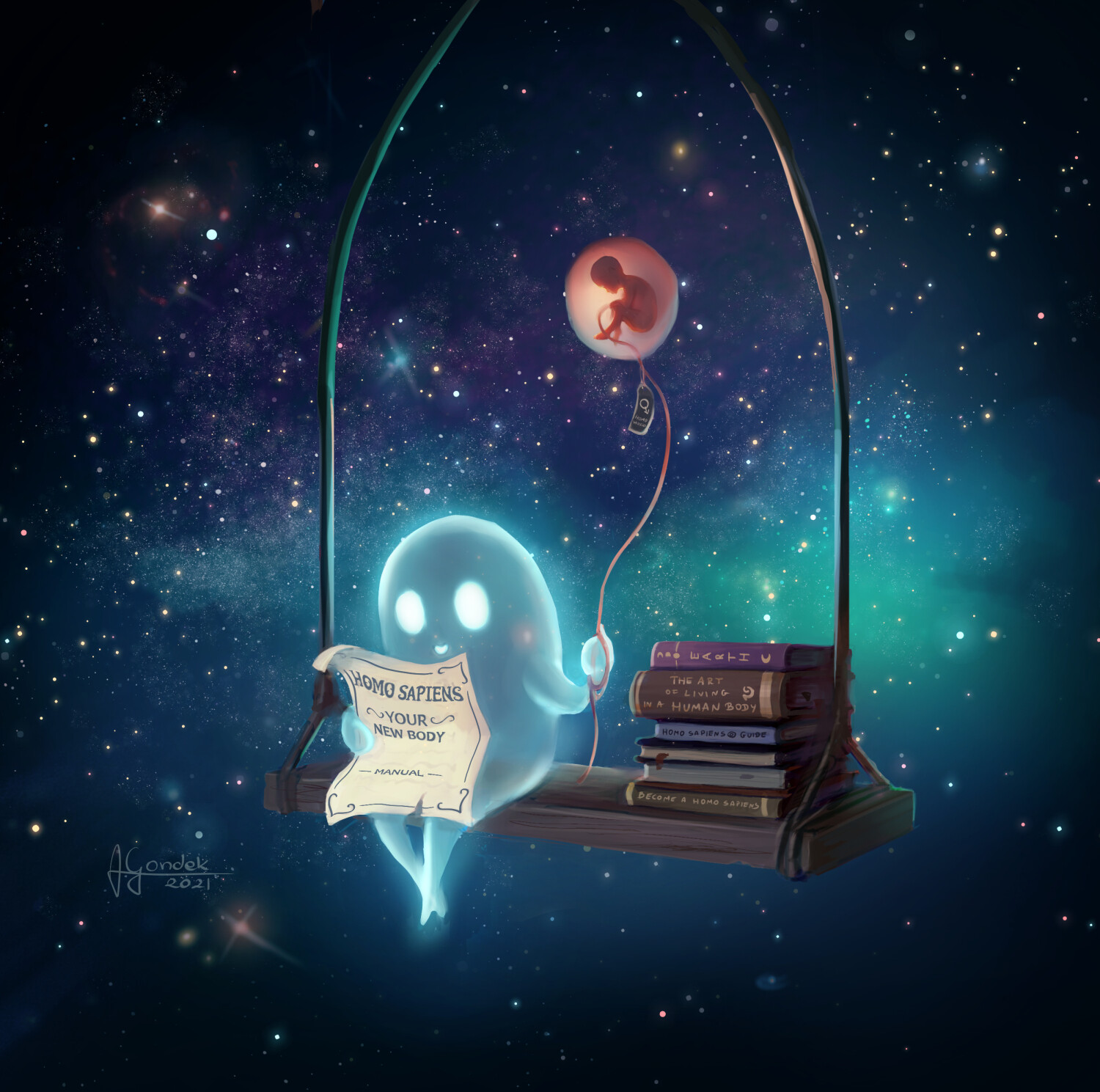This captivating illustration features a small ghost with a bulbous body, seamlessly blending its head, neck, and torso into one unified form. The ghost emits a soft blue glow, accentuated by its luminescent white eyes. It is perched on a makeshift tree swing, composed of a simple wooden board suspended by cables or possibly wooden bars that converge above. 

Beside the ghost on the swing, there is a neatly stacked pile of books, totaling around eight in number. Titles such as "The Art of Living in a Human Body" and a book about death are discernible among them, hinting at themes of existence and mortality. Grasping the book "Homo sapiens: Your New Body" in its right hand, the ghost appears to be engaged in a contemplative exploration of human life.

In its left hand, the ghost holds a unique helium balloon, tethered not by a conventional string, but by an umbilical cord. Within this pink, translucent balloon, a fetus is clearly visible, positioned sideways as it continues to develop. This surreal image suggests the ghost's involvement in nurturing the fetus, preparing it for a human form.

The background is an ethereal expanse of space, with stars and nebulae creating a cosmic setting. The tree from which the swing hangs seems to float in this void, adding to the otherworldly ambiance. The illustration is signed by Jay Gondek, dated 2021. Through this intricate and imaginative depiction, the artwork conveys a profound and enigmatic narrative of life, death, and transformation.